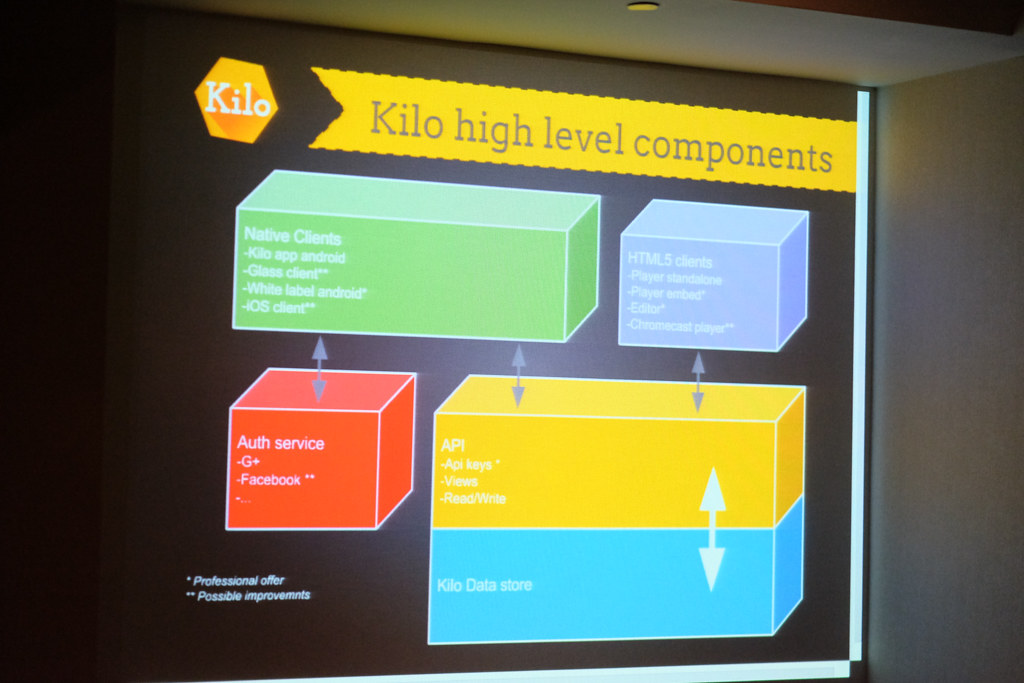The image showcases a PowerPoint slide projected onto a wide, rectangular screen, revealing a detailed graphical layout against a black background. In the upper left corner, an orange hexagon prominently features the word "Kilo" in white font. Adjacent to the hexagon, a yellow ribbon-like banner spans the top of the slide, ending in a triangle that mimics a ribbon edge, with the text "Kilo High Level Components" in gray font.

Below this, the slide displays four rectangular prisms, outlined in white and filled with various colors: green, purple, red, blue, and yellow, each containing lists of terms written in white. The green rectangle lists items like "Native Clients, Kilo App Android, Glass Client, White Label Android, iOS Client." The purple rectangle includes terms such as "HTML5 Client, Player Standards, Player Embed, Edit, Chromecast Player." The red rectangle mentions "Ops, Service, G+, Facebook" and features two stars. The blue and yellow rectangle, split into two halves, has the text "Kilo Data Store" on the blue half with an accompanying arrow pointing downwards, suggesting a flow or relationship.

The screen is positioned on the right side of the image, with the ceiling and adjacent wall visible around it, highlighting the mounted display's setting. The overall layout appears to depict some kind of flowchart, illustrating the interconnected components with gray arrows indicating their relationships.